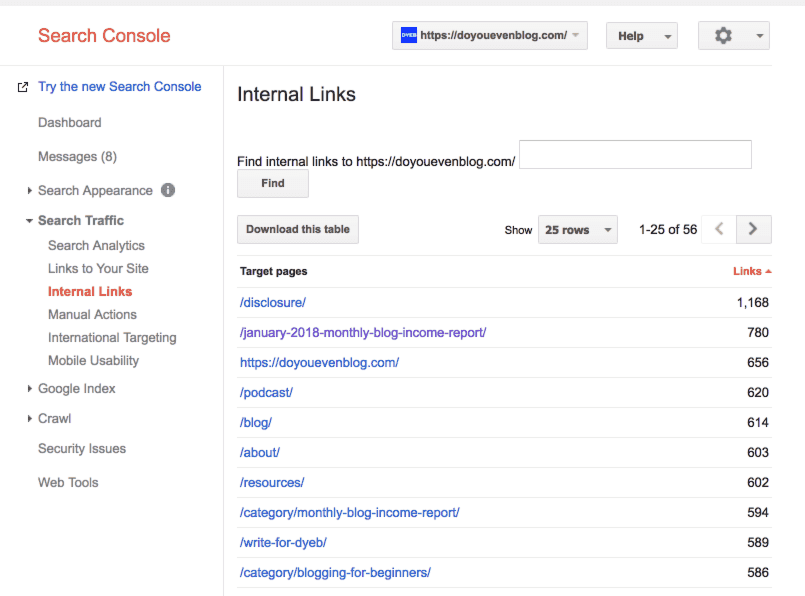This is a screenshot of a Google Search Console interface, displaying various features and metrics for the website "DoYouEvenBlog.com." In the top left corner, the label "Search Console" is prominently displayed in orange text. Just below this, an invitation to "Try the new Search Console" is noted. The interface includes multiple tabs: Dashboard, Messages (indicating 8 unread messages), Search Appearance, Search Traffic, Search Analytics, Links to Your Site, Internal Links, Manual Actions, International Targeting, Mobile Usability, Google Index, Crawl, Security Issues, and Web Tools.

In the top right corner, a link to the website DoYouEvenBlog.com is visible. Beneath this, the section titled "Internal Links" is highlighted, with tools allowing users to find and download internal link data. The current focus is on target pages showing internal link counts, which include entries such as "Disclosure," "January 2018 Monthly Blog Income Report," among others, with the number of links to each target page listed on the right side.